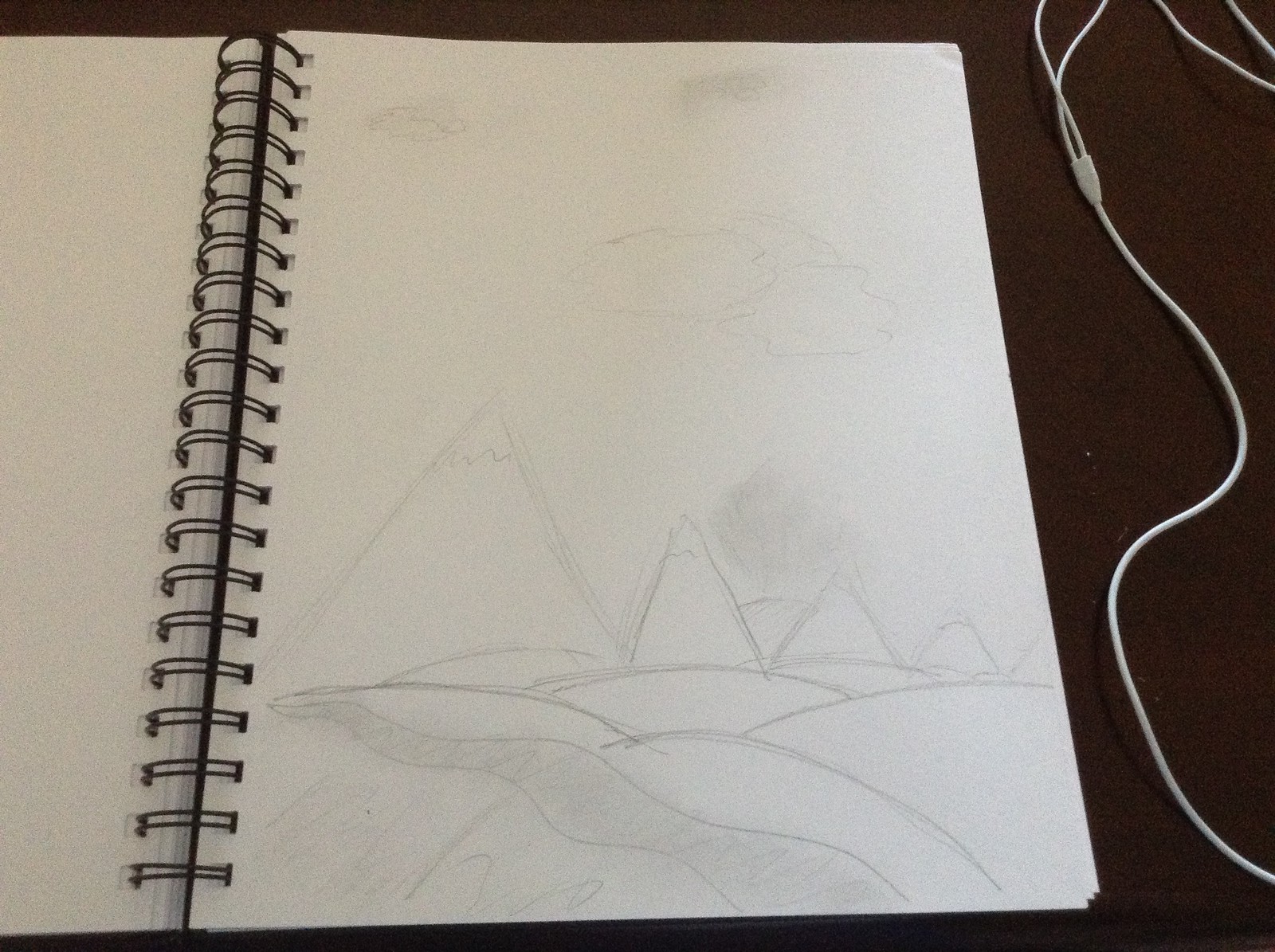In the background, there's a brown wooden desk. A white electrical cord, possibly for earbuds, is visible on the desk. To the left of the desk lies a spiral notebook with plain, white, unlined pages. The notebook showcases a pencil sketch featuring mountaintops with the sun peeking over them and light clouds in the sky. The drawing also includes rolling hills and a dark spot resembling a small lake, all delicately rendered in light pencil.